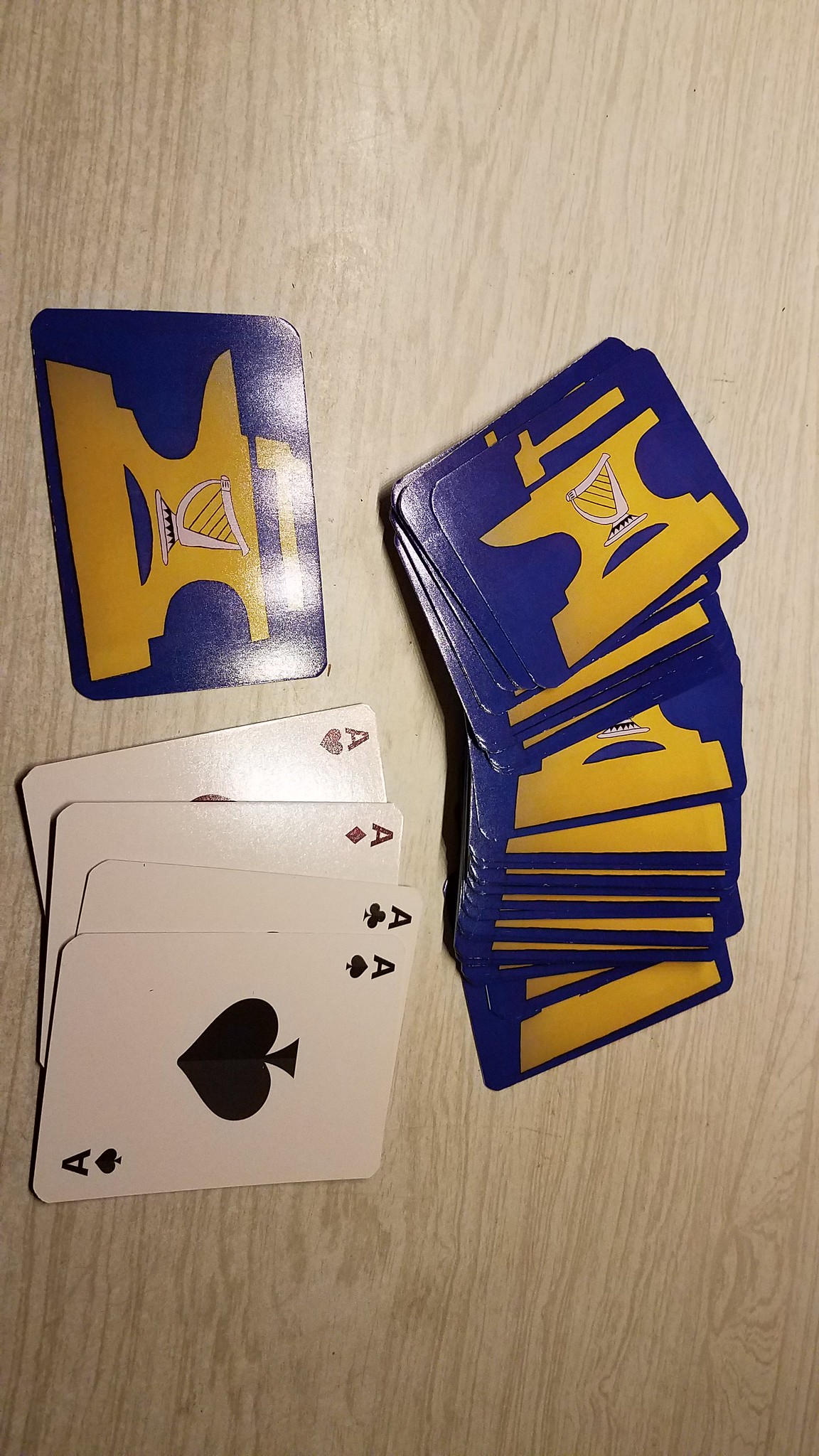This image captures a light-colored wooden table, marked with dark lines that create a textured pattern. At the center of the table lies a disorganized deck of playing cards. The card backs are predominantly purple with a hint of blue and feature a distinctive, intricate design: a yellow anvil at the base, topped by an axe, and crowned with a harp. Alongside this deck, there are four aces prominently positioned. The spade is the most visible, with just the small upper symbols of the heart, diamond, and club peeking out. Additionally, one card lies face-down next to the aces, while the remaining cards are spread out in a fan-like arrangement, giving a glimpse of the set’s pattern and design.